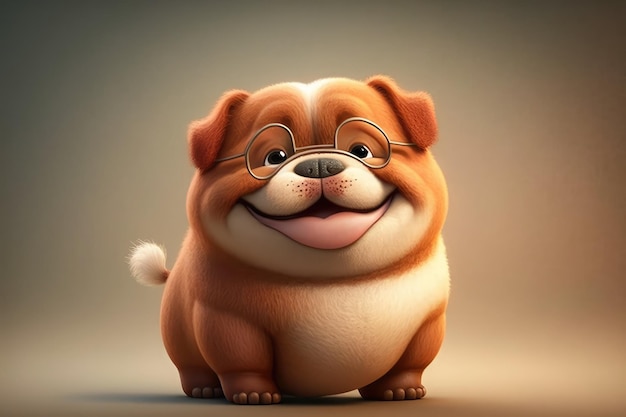This AI-generated digital illustration features a cartoonish, overweight dog positioned front and center against a nondescript, fading gray background. The dog, rendered in shades of orange, reddish-brown, and tan, exudes happiness with a broad, toothless smile and a prominent, pinkish human-like lower lip. His snout and lower jaw are white, as are a tuft of fur at the end of his little tail, and his chest, which transitions into the rest of his coat. His round, silver wire-rimmed glasses perch on his pushed-up nose, which is decorated with freckle-like whisker spots. The dog’s floppy ears fold forward, almost covering his face, and his short, stubby legs barely support his generous midsection. Paws and legs hit the ground at the same spot, and his cheerful demeanor is enhanced by his big smile and diminutive, stubby tail poking out behind him.